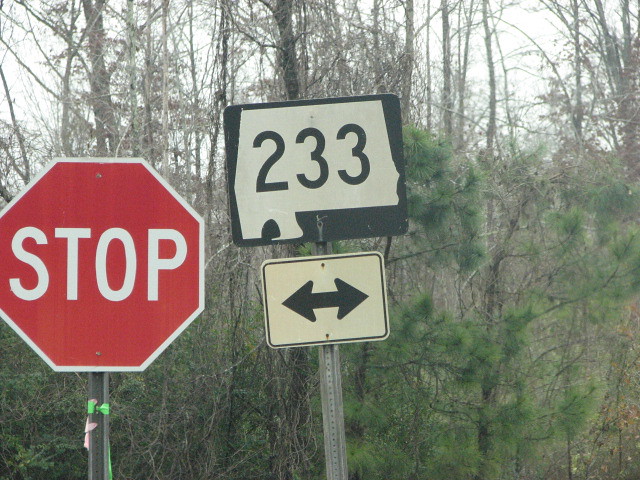In this detailed photograph taken during the day, we prominently see two road signs mounted on gray metal posts standing on the side of a road. The leftmost sign is a red octagon stop sign, with a white border and bold white text reading "STOP." To its right, another sign features two placards. The top placard is a black and white square with the numbers "233," though somewhat deformed. Below it, a rectangular white sign with black border and text displays arrows pointing both left and right. Surrounding these signs is a tree-lined background, with a mix of trees - some barren or with brownish leaves, and others full and green. The bright, white sky gleams through the sparse treetops, creating a contrast against the dense foliage below.